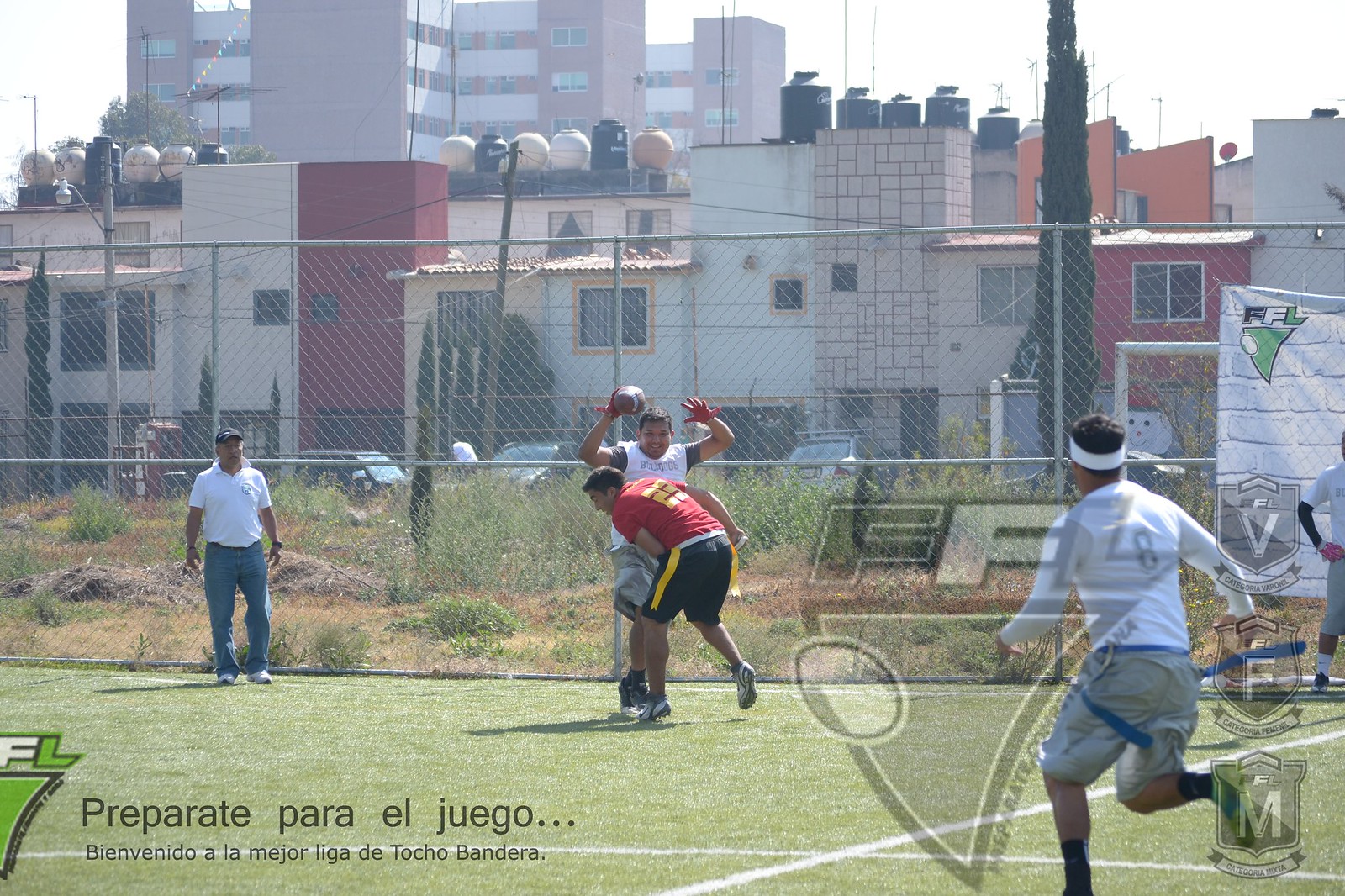The photograph captures a casual game of American football with four players in an urban park setting. The players are on a green field, possibly artificial turf, marked with white lines that form a cross, suggesting it might be a multi-purpose field rather than a traditional football field. On the left, an older man in jeans, a white polo, and a hat spectates from the background. The other three players are actively engaged; one holding a football in a white jersey and shorts, another approaching him dressed in red, black, and yellow, while the third runs in a white shirt and gray shorts on the far right. The park is enclosed by a tall silver chain-link fence.

Beyond the fence, there is a vibrant residential area with colorful apartment buildings; some are red, others white with yellow-trimmed windows. Further behind, several taller structures, possibly offices or hospitals, dominate the skyline. The lower left of the image features the text "Preparate para el juego, preparing for the game" and "Bienvenido a la Mejor Liga de Tocho Bandera," suggesting it's an advertisement for a touch football league. A watermark resembling a checkmark and an "M" logo, possibly for a team, are visible in the lower right corner.